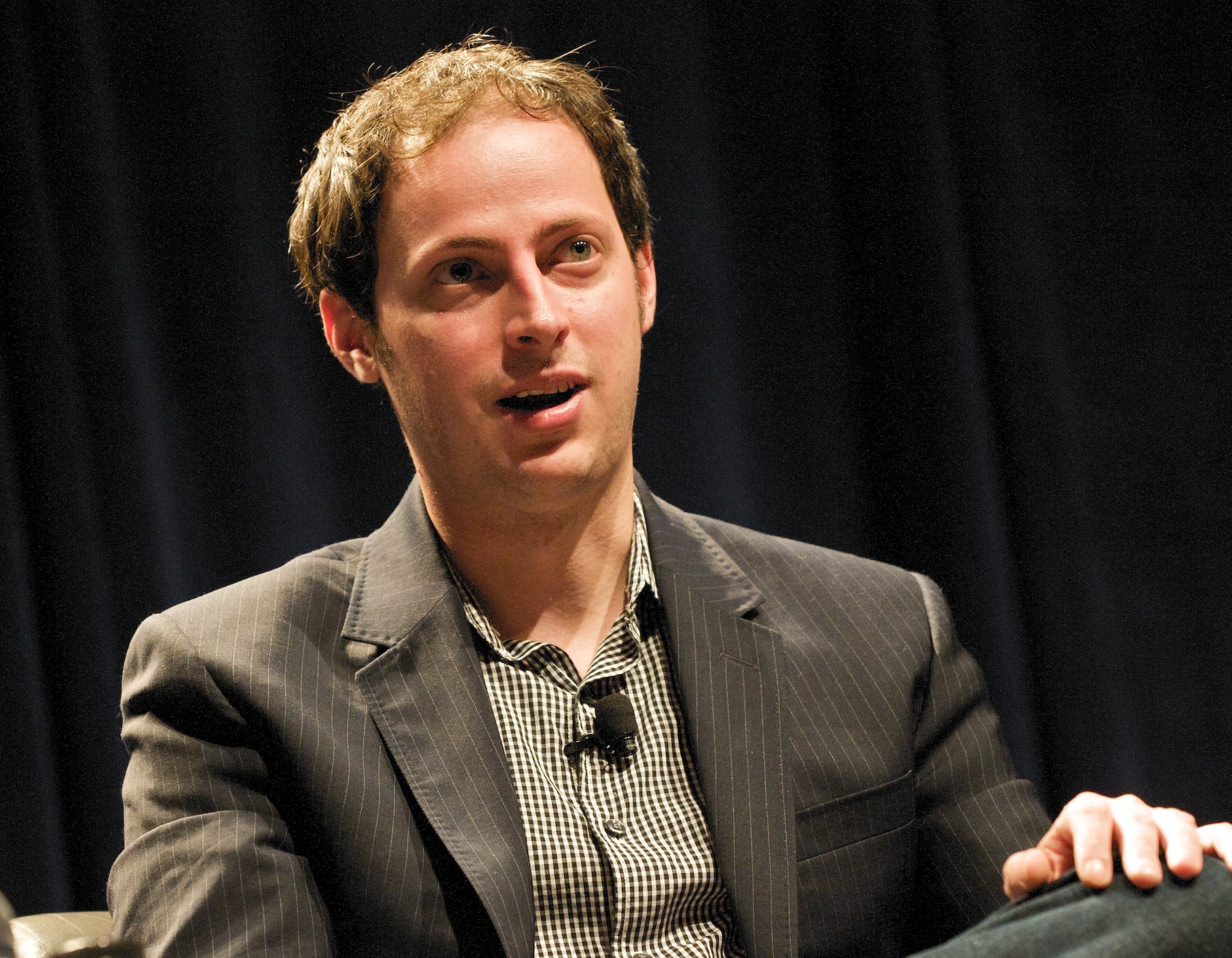A middle-aged white man, likely in his 40s or 50s, is seen sitting on a chair against a backdrop of dark navy blue or black curtains, suggesting the setting could be an interview or conference. Dressed in a black suit paired with a black and white checkered shirt, he is not directly facing the camera but is turned towards the audience, engaged in speaking. His facial expression reflects a blend of nervousness, excitement, and confidence. While he is evidently a public figure, his exact identity is not immediately recognizable.